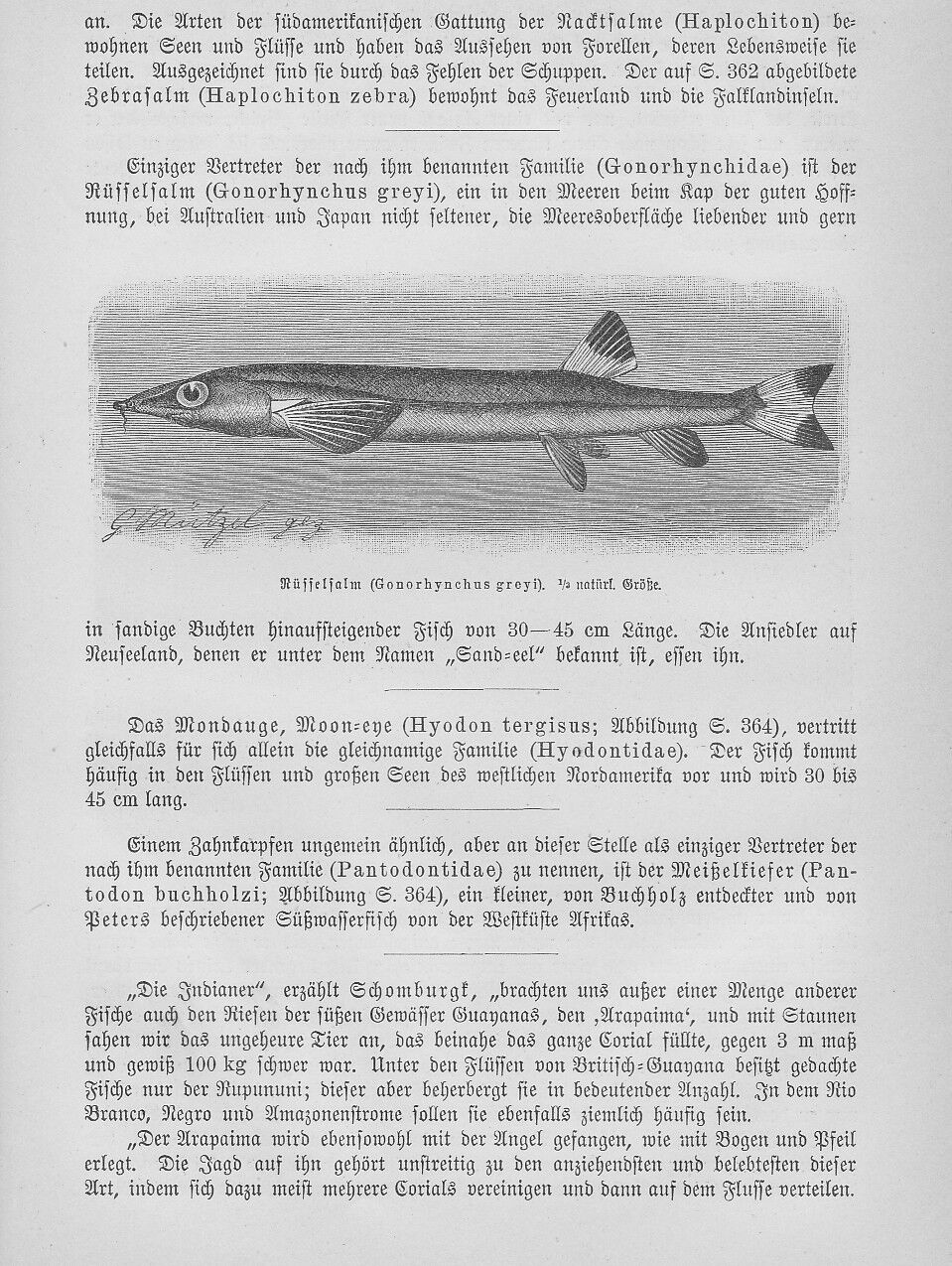The image depicts a rectangular page from a book, with the length of the left and right sides being twice that of the top and bottom. The light gray page features multiple lines of black text, all in German, making most of it unreadable. The text is segmented by thin black lines separating different ideas or passages. Prominently featured towards the top center of the page is a detailed black and white sketch of a long-bodied fish. The fish has large eyes that dominate its head, whiskers at the front, a single small fin on its upper back, two fins on its sides, three fins underneath, and a sharply pointed tail fin. Below this finely drawn fish, there is a small signature on the bottom left. The layout includes several paragraphs – approximately seven or eight – above and below the fish, separated by a thin black line, set in a fancy font. The presence of the fish and the text suggests that this page could be from a book or a magazine, potentially about fishing.